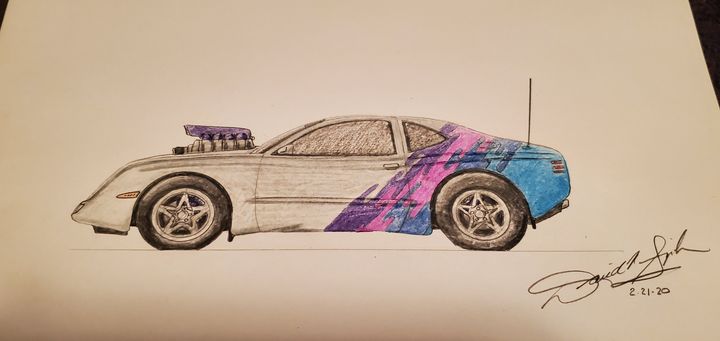This image depicts a detailed, hand-drawn representation of a sports car by an artist named David, with his signature and the date "2-21-20" in the bottom right corner. Rendered primarily in graphite pencil, the car showcases a sleek, two-door design with large, black tires featuring five-star rims. The drawing is done on white paper, with the car oriented horizontally and viewed from the left side. The car's aerodynamic contours and tinted windows are meticulously shaded in grayscale.

The front section of the car, which covers the hood and extends to the front doors, remains in a black-and-white gradient, while the rear end is distinguished by vibrant splotches of color. These colors—primarily purple, pink, and blue—are artistically streaked diagonally from the back bumper to the middle of the car. Notably, a purple-colored intake or exposed engine component protrudes from the hood, adding to the car's high-performance aesthetic. Furthermore, there's an orange light near the front wheel, complemented by fine detailed lines, enhancing the car's realism and dynamic appearance. 

Overall, David's drawing masterfully combines detailed pencil shading with vivid color accents, creating a visually striking and lifelike depiction of a customized sports car.